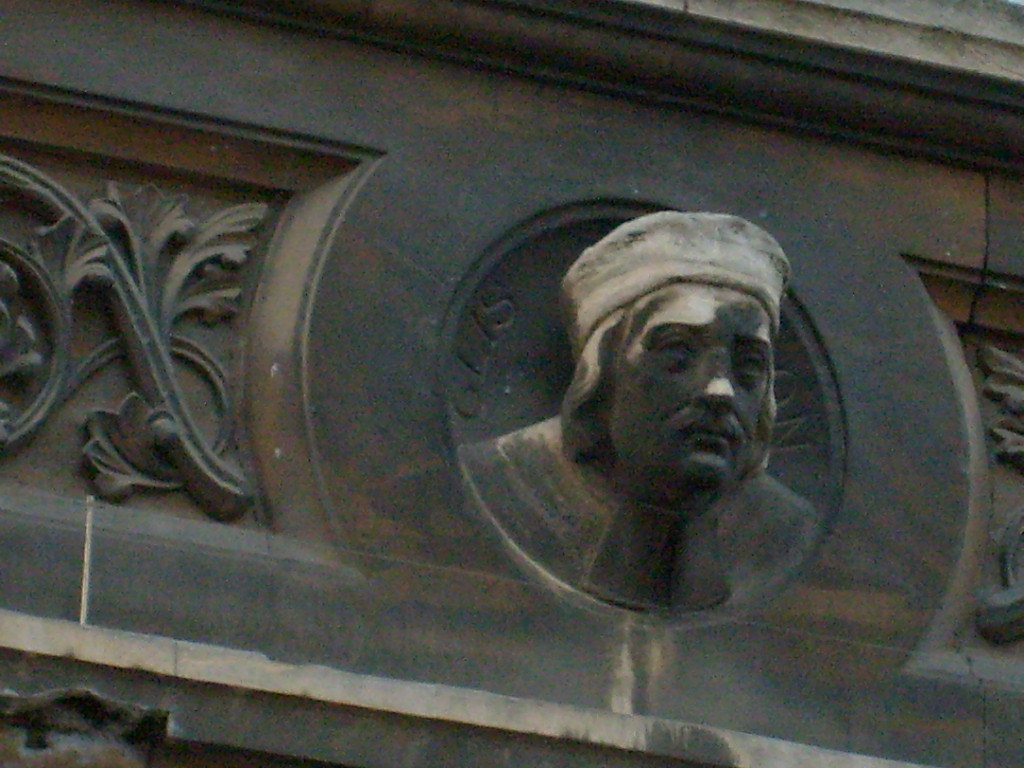This image captures a rectangular outdoor photograph focusing on a bas-relief carving on the side of a dark stone building. The carved stone wall, dark brown to black in color, features a contrasting white ledge running across the bottom, creating an indented or concave effect. Central to the image is a smooth, intricately carved circle resembling an "O," from which a male figure’s head protrudes. The figure, rendered in a gray hue, wears a distinct flat, round hat that flushes across his forehead and crowns the top of his head. His somber face is detailed with a straight nose, potential mustache, and long hair cascading to his shoulders and over his ears. There is some inscribed text around the concave circle, challenging to decipher but possibly reading "Gust U.S." or similar initials. Flanking the central figure, faint carvings of leafy vines weave through the stonework, adding texture and interest to the wall. Sunlight and shadows play across the relief, enhancing the intricate details of the carving and the building's stone texture.